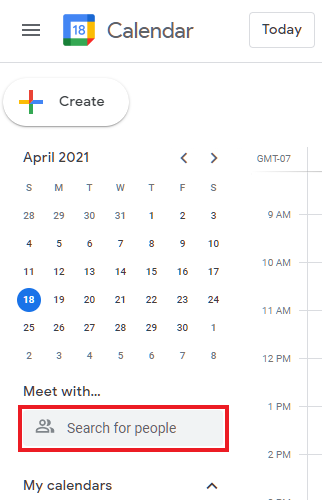The image depicts a Google Calendar interface, predominantly showcasing the month of April 2021. On the top left corner, there's a hamburger menu icon. To the right, an 18 is enclosed within a box, colored in Google's signature palette of red, blue, green, and yellow, with the box's bottom-right corner clipped off. Next to the box, the word "Calendar" is prominently displayed. 

Situated nearby are tabs labeled "Today" and "Create," both in Google colors, with the "+" symbol indicating the creation of new events. In the main section of the interface, the calendar dates for April 2021 are visible, with Sunday the 18th highlighted. 

Below the dates, a "Meet with..." search box allows users to look up people. Underneath, a tab labeled "My calendars" includes a drop-up arrow for additional options. 

On the far right side of the screen, a vertical time grid is visible, displaying time slots starting from 9 a.m. to at least 2 p.m., though the remainder is cut off. The timezone displayed is GMT -7. 

Overall, the image is a clear representation of a Google Calendar page set to April 18, 2021.